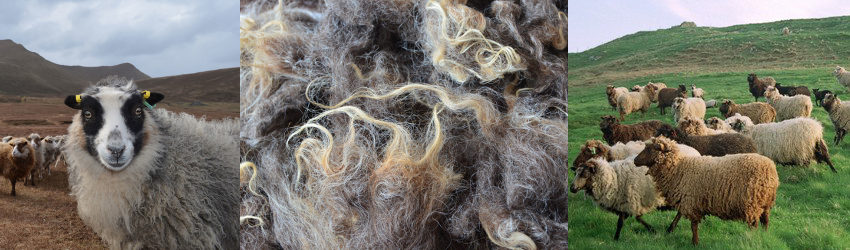This is a collage comprising three outdoor photographs taken during the daytime, showcasing various aspects of sheep in their environment. In the leftmost image, a sheep stares directly at the camera with an endearing expression. This sheep features whitish-gray wool with a white stripe down the center of its face surrounded by black around both eyes and black ears adorned with orange identification tags. The background reveals additional sheep scattered about in a barren, brownish field, set against a backdrop of distant mountains and a cloudy sky. The center photograph offers a close-up of tangled and matted sheep wool, displaying an intricate mix of gray, white, brown, and tan fibers, suggestive of the natural texture and coloration of sheep fleece. In the rightmost image, a lush green hillside comes to life with around 15 sheep grazing and moving about. Each sheep varies slightly in color, ranging from cream and light tan to darker brown shades. This scene, bathed in sunlight, highlights the wool’s reflective properties, adding a vibrant, lively element to the composition. Together, the images capture an array of details, from the intimate features and markings of an individual sheep to the collective behavior and diverse wool textures of a flock in different settings.